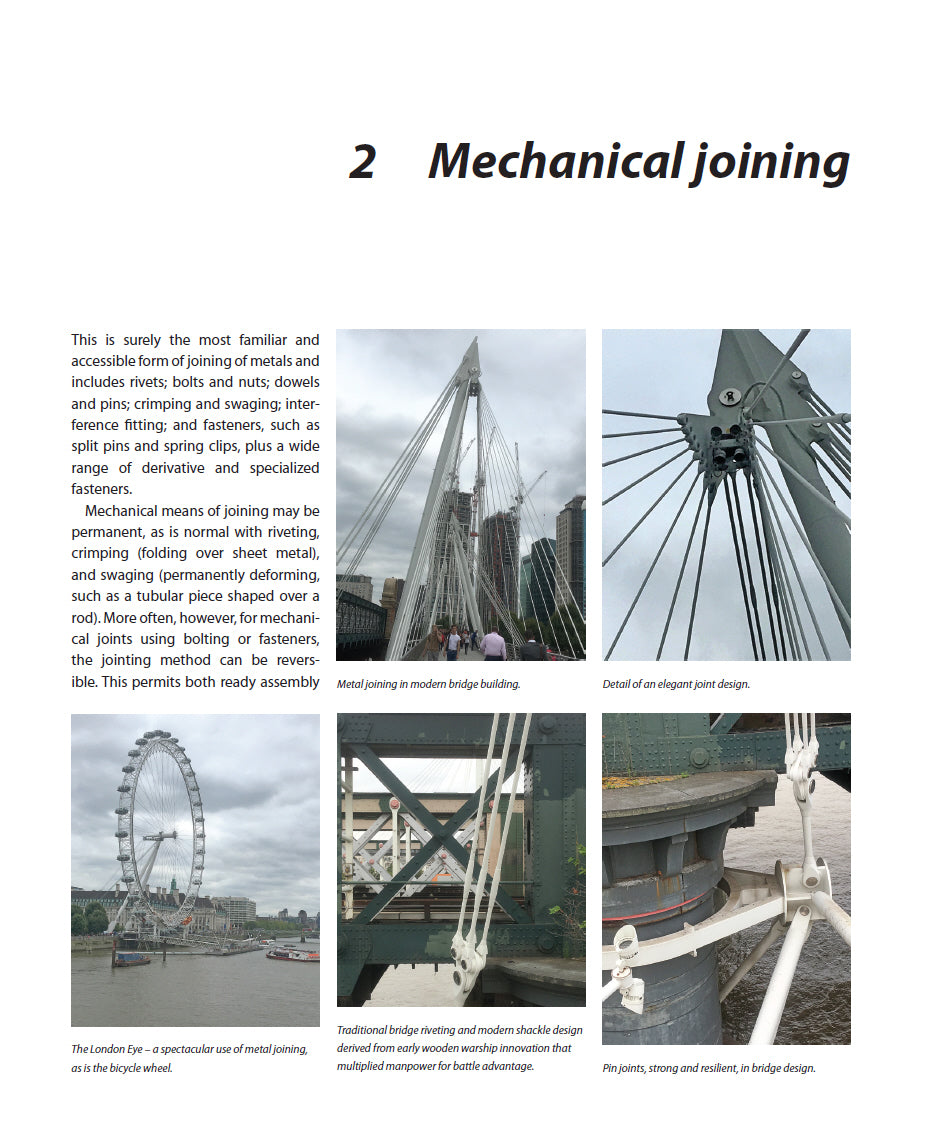Caption for the image:

The image is a detailed snapshot from an informational book, focusing on the methods of mechanical joining. The heading at the top of the page, written in bold black text, reads "Two Mechanical Joining." Below the heading are five images, arranged in two rows: two images at the top and three at the bottom. The first picture at the bottom row has an accompanying caption that reads: "This is surely the most familiar and accessible form of joining of metals, including rivets, bolts and nuts, dowels and pins, crumpling and swaddling, interference fitting and fasteners, such as split pins, spring clips, plus a wide range of derivative and specialized fasteners." Other images under this include notable examples of mechanical joining: one labeled "The London Eye", showcasing an impressive use of metal joining in its construction, and another featuring a bicycle wheel. There is also an image of white bolts with the caption "10 joints, strong and resistant," used in bridge design, illustrating the importance of robust mechanical joints in structural engineering.